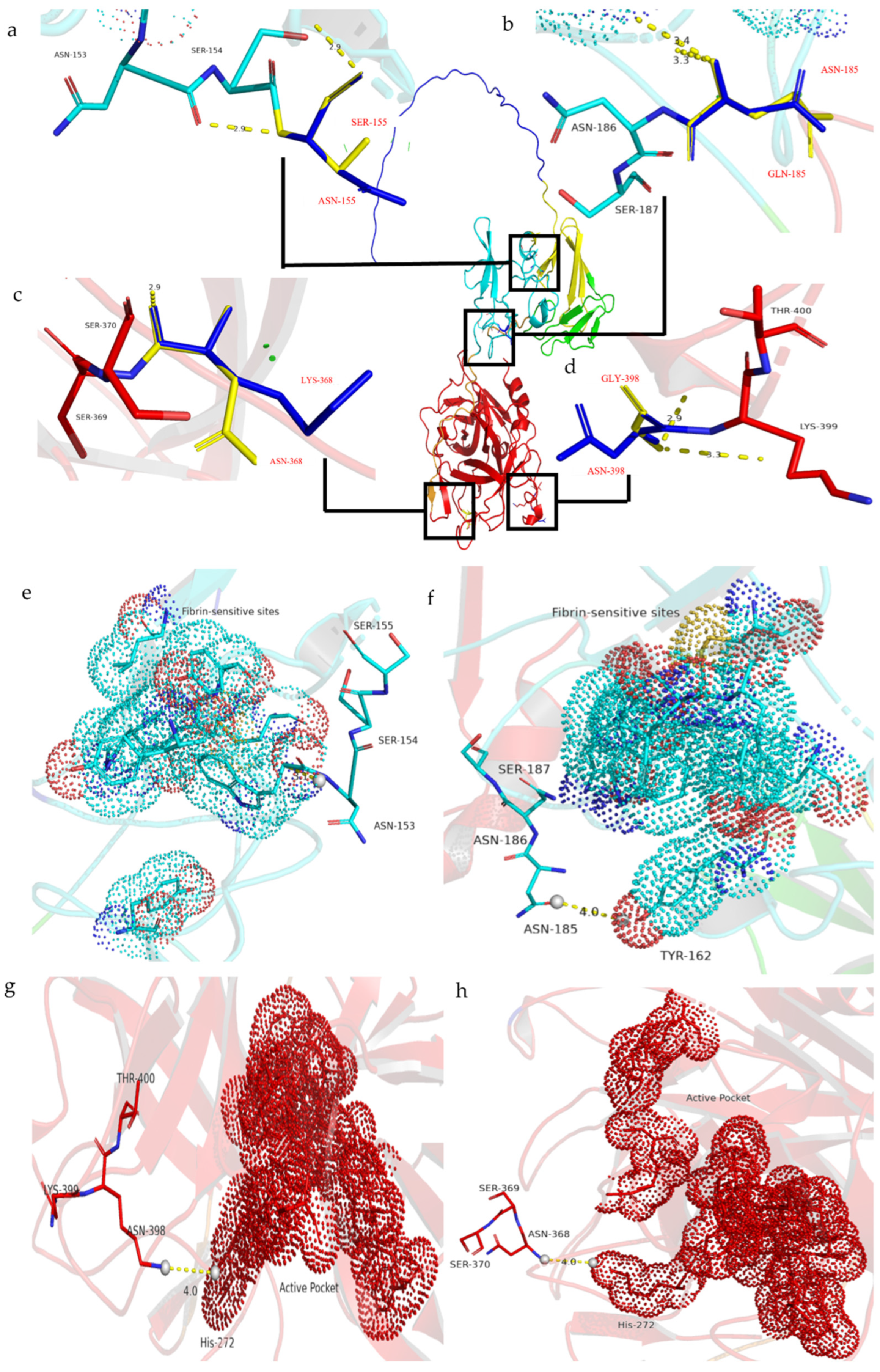This detailed and vibrant vertical image appears to be a scientific diagram, possibly from a science book, explaining molecular structures and interactions. It features eight sections labeled A through H, each demonstrating different aspects related to molecule assembly or structure. The image includes several colors such as blue, turquoise, yellow, and red, with many molecules having components in these hues. 

The upper four diagrams (A-D) display linear structures with intersecting shorter lines, resembling strings of DNA or molecular strands, and include labels with specific letters and numbers such as ASN-153 and SCR-154. These diagrams use colors like teal green and bright red, with some blue and yellow edges.

The lower four diagrams (E-H) shift to more complex, blob-like shapes akin to amoebas or cells. The drawings feature circly blobs of dots surrounding central lines and are primarily illustrated in blue tones with the addition of red in the bottom rows. The two sections directly below the molecular strands retain similarities but exhibit brighter and more pronounced red hues. Overall, the detailed depiction using varied colors and intricate labeling aids in visualizing different molecular forms and their interactions.